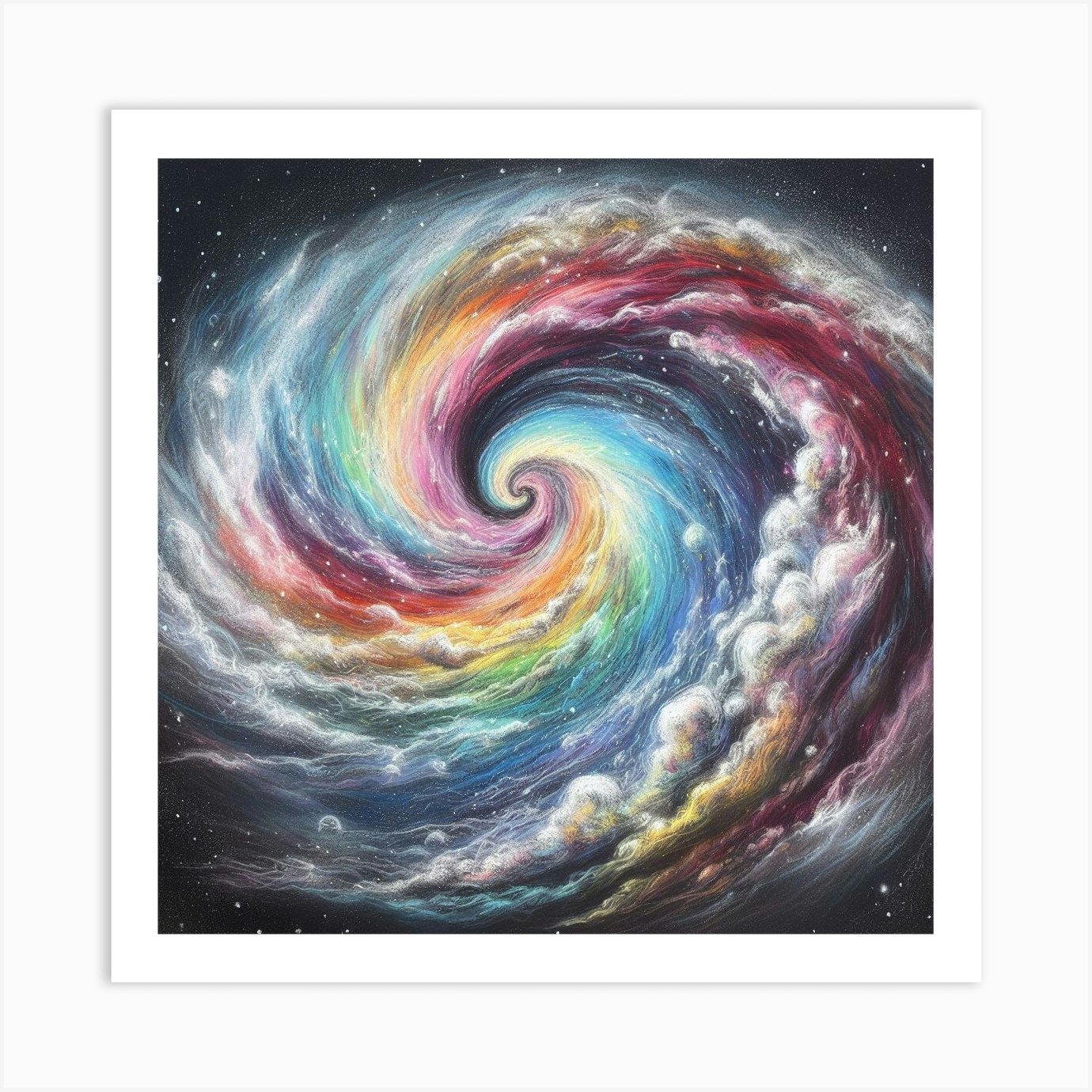The image is a detailed artistic depiction of a galaxy or a cosmic swirl, printed and displayed on a wall. The focal point of the artwork is a mesmerizing spiral that starts at the center and expands outward, featuring a spectrum of rainbow colors. Hues of pink, red, orange, yellow, and green blend seamlessly with white swirls, which appear to be clouds, smoke, or stars, adding depth and dynamism to the scene. The swirl, which moves counterclockwise, is intricately drawn with colored pencils or possibly pastels or chalk. Surrounding the vibrant core, the corners of the image are cloaked in blackness, adorned with white specks resembling distant stars. The overall composition captures a magical, ethereal quality, presenting an enchanting vision of the universe that is both detailed and pleasing to the eye.